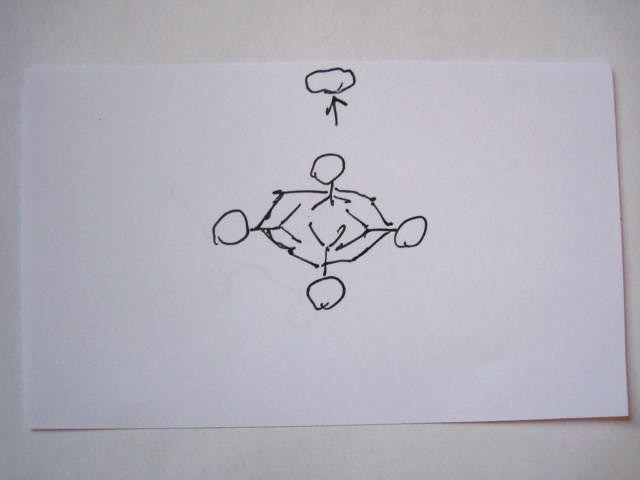The image showcases a surface that appears to be either a light gray or slightly off-white wall, table, or counter, with a subtle watercolor-like pattern. Placed on this surface is a blank white horizontal rectangular piece of paper. Centered at the top middle of the paper, drawn in black marker, is an irregular, slightly oblong shape with an upward-pointing arrow underneath it. 

Positioned precisely in the very center of the paper is a hand-drawn octagonal shape. This octagon is adorned with four protrusions extending outward, each ending in a small circular shape. The central structure is designed to evoke a three-dimensional effect, though somewhat imperfectly. The intent and effort to give depth to the drawing are evident, despite not being entirely convincing. The purpose of this drawing remains unclear, as no additional context or enhancements are present on the paper.